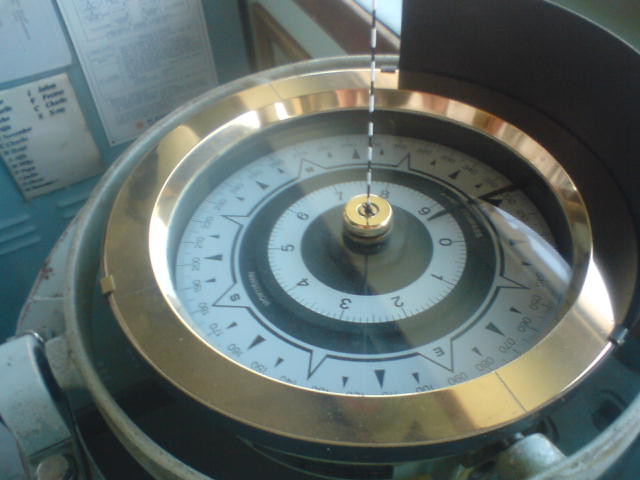In this image, we see a well-worn gauge or meter mounted centrally. The gauge is encased in a light gray frame, dotted with patches of brown rust, particularly noticeable on the left side and the bottom right corner. Surrounding the gauge is a shiny, glossy, gold frame that adds a striking contrast to the aged appearance of the instrument. The gauge features a white face displaying black numbers and symbols, with a prominent black-and-white pointer at its center.

To the top left of the gauge, there are three blue lockers, each with three ventilation slots on their doors. Affixed to these lockers are several white papers: two small documents in the upper left corner, and a larger poster-like piece in the top center. The papers are white with black text, though the exact content is not discernible.

Additionally, in the top center section of the wall, brown trim creates a border, extending around what appears to be a picture frame directly above the gauge. This framing detail adds an element of orderly structure to the otherwise industrial setting.